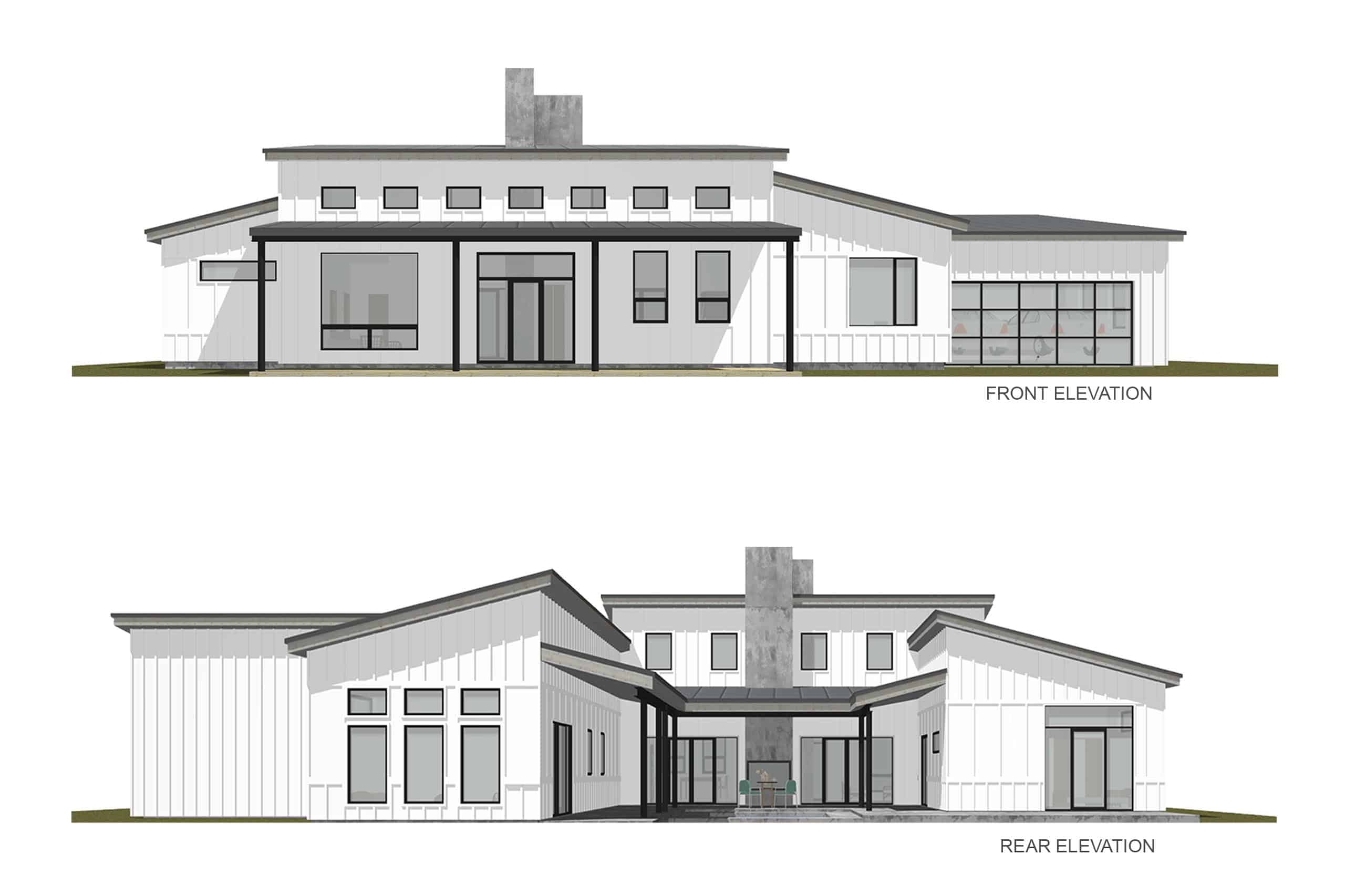The image showcases detailed black and white architectural drawings of a modern, two-story house, depicting both its front and rear elevations. The drawings are in gray scale and are stacked vertically against a pure white background, accentuating the sophisticated and sleek design of the house. The top illustration, labeled "Front Elevation" in the bottom right, features a spacious front facade characterized by a large porch overhang, a prominent chimney, and is embellished with numerous windows — seven on the upper level alone. There are two wings extending from either side of the house, with one wing incorporating a see-through garage door, hinting at a car inside. Meanwhile, the lower illustration, labeled "Rear Elevation," reveals an expansive patio area that is integrated with the chimney. The rear of the house includes additional features such as glass doors, which are likely sliding, and multiple windows across the top story and the wings, enhancing natural lighting and providing ample storage space.